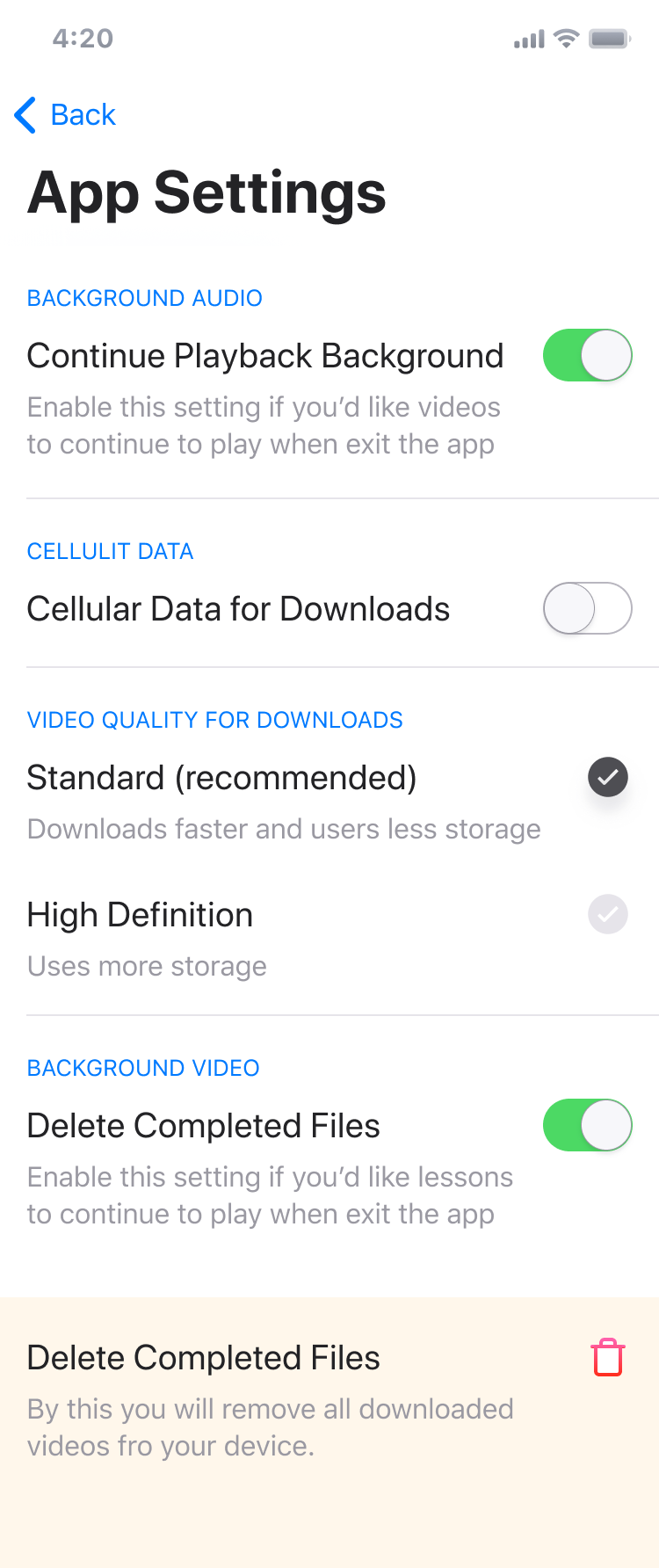This is a detailed screenshot of a smartphone displaying the app settings menu. At the top-left corner, small gray letters indicate the time as 4:20. Adjacent to the time, the display shows the Wi-Fi signal icon, mobile data signal strength, and battery percentage indicator.

Directly below, in blue, there is a left-pointing arrow accompanied by the word "Back." Prominently displayed in bold black letters is the title "App Settings."

Under the title, the menu begins with "Background Audio" written in small blue letters, followed by the description "Continue playback in background." This option features a green toggle switch that is slid to the right, indicating it is enabled. 

Next, the section labeled "Cellular Data" is introduced in blue letters, with "Cellular Data for Downloads" written in black underneath. A slider beside this text is positioned to the left, showing that it is turned off.

Further down, there is a setting labeled "Video Quality for Downloads" in blue. Directly below, in black, it states "Standard (recommended)" with a checked circle next to it, signifying the selected option. Another option "High Definition" is listed next, also in black, but its associated circle is grayed out, indicating it is not selected.

Following that, "Background Video" is in blue letters with "Delete Completed Files" in black letters underneath. This includes a green toggle switch set to the right, signifying it is active.

Finally, at the bottom of the screenshot, the phrase "Delete Completed Files" appears again alongside a red trashcan icon.